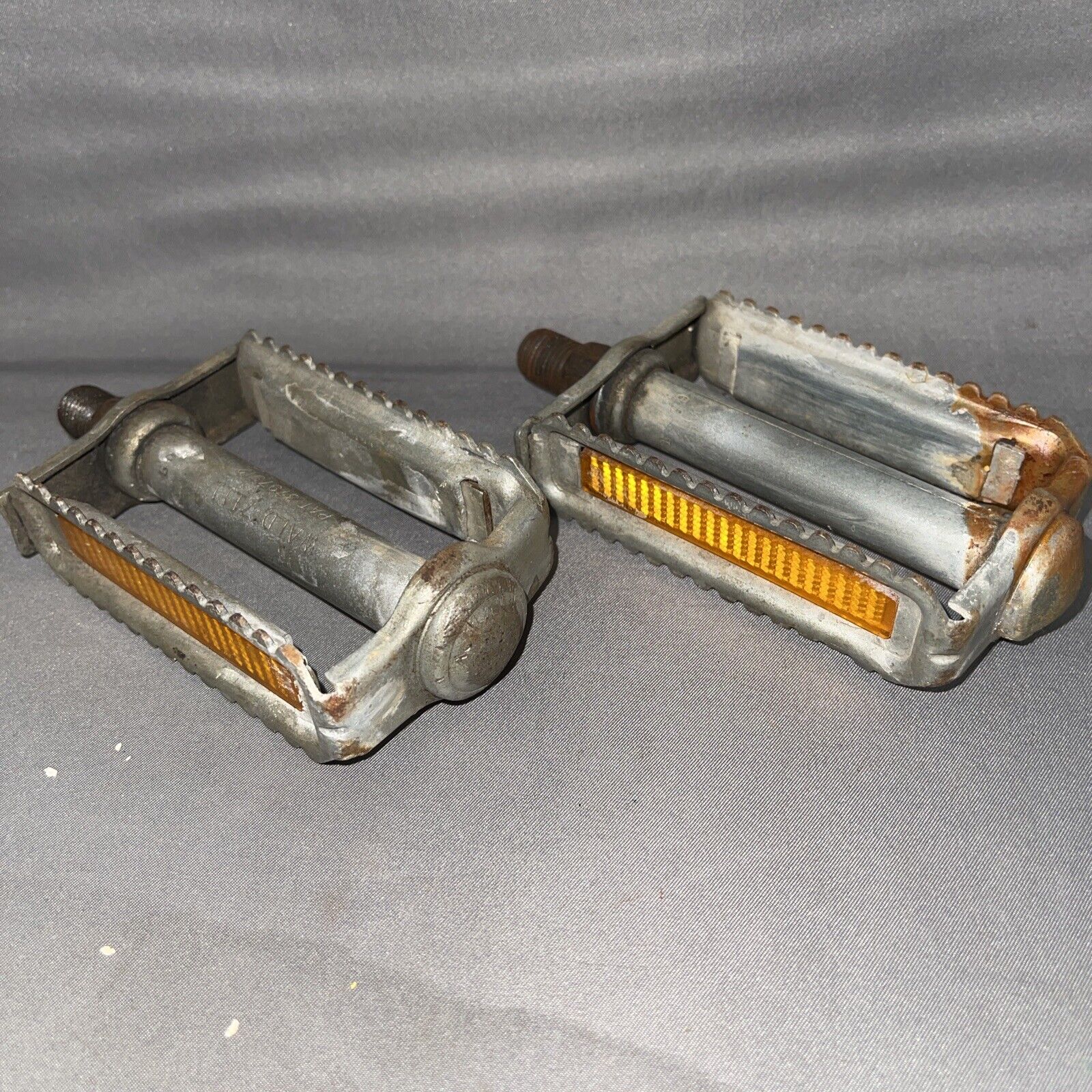The image features two weathered bicycle pedals laid out on a dark gray cloth background. These rectangular pedals, angled slightly downward to the right, exhibit signs of wear and light rust. Each pedal has a central metal cylinder with bolt threads protruding from the left side, and reflective yellow-green plastic strips are installed on the sides for visibility. The outer edges of the pedals are equipped with teeth designed to provide grip for the feet. Despite their worn appearance, they remain mostly intact and appear to have been recently removed from a bicycle.